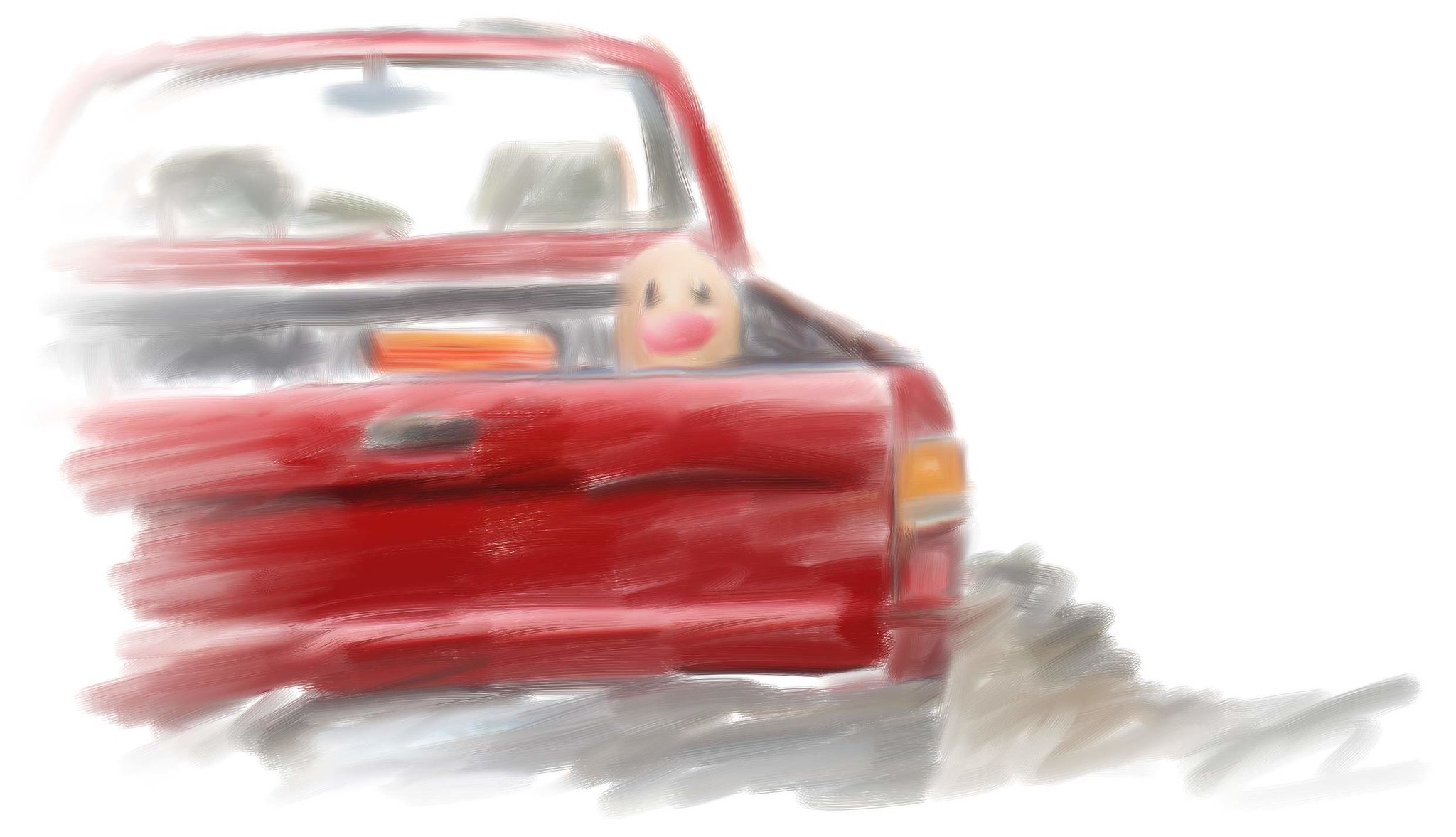This image appears to be a painting or drawing, possibly done in watercolor or marker, depicting a red pickup truck driving away, set against a stark white background. The truck is primarily positioned from the middle to slightly right of the image and extends towards the left. The bed of the truck is open and appears gray, featuring a red tailgate with a white or gray latch. The tailgate handle is also gray. Yellow turn signals and red brake lights are visible on the right-hand side of the truck. In the bed of the truck, there is an orange rectangular object situated against the front.

A striking feature within the truck bed is an unusual flesh-colored oval shape resembling a face, with large pink lips and two dark, feathery circles for eyes. This face peers towards the back of the truck, adding a whimsical element to the artwork. The rear window of the truck reveals part of the vehicle's interior, including the tops of the front seats and a rearview mirror positioned centrally.

Along the bottom of the image, there's a distinct gray swirling or shading that might represent the ground, road, or possibly smoke emanating from the truck’s exhaust. This gray area extends from the bottom right and continues across to the left side of the image.